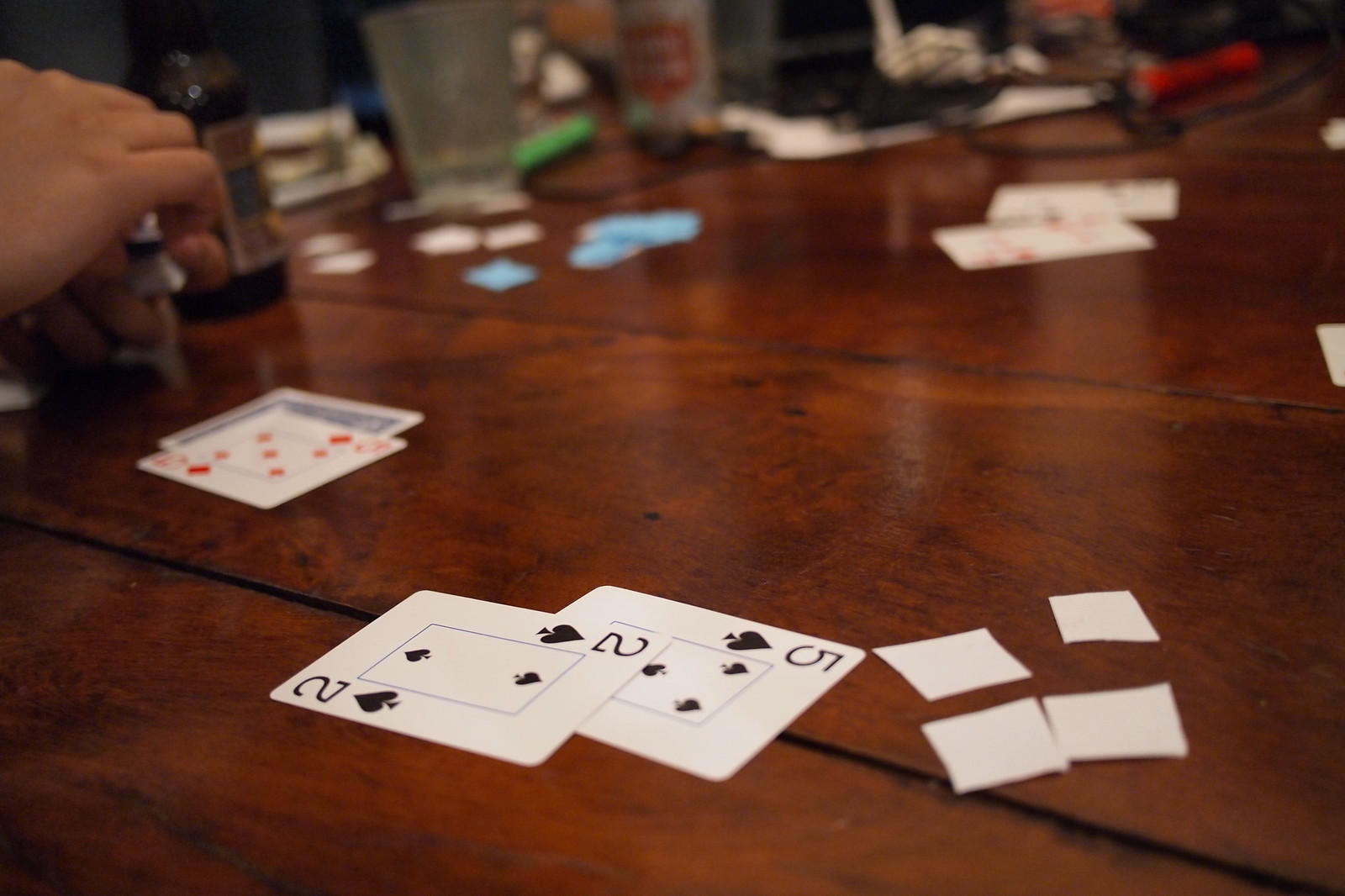This photograph, taken with a high aperture setting likely around f/1.4, captures a richly detailed dining room scene centered around a walnut table with a distinctive black stripe running diagonally from the bottom right to near the center left of the frame. Emerging from the top left corner is a partially visible hand. The focus of the image is on a pair of playing cards in the center near the bottom—the two of spades resting atop the five of spades. To the right of these cards are four small white squares, resembling sugar packets, scattered on the table. Just below the hand, the five of diamonds can be seen with another card flipped over beneath it. The background is a soft blur, featuring additional playing cards that are too indistinct to be identified. There appears to be miscellaneous clutter and more small packets, including some blue ones, possibly items like chips, though they are too out of focus to determine. The walnut table itself has a glossy finish, showcasing its intricate burl pattern.